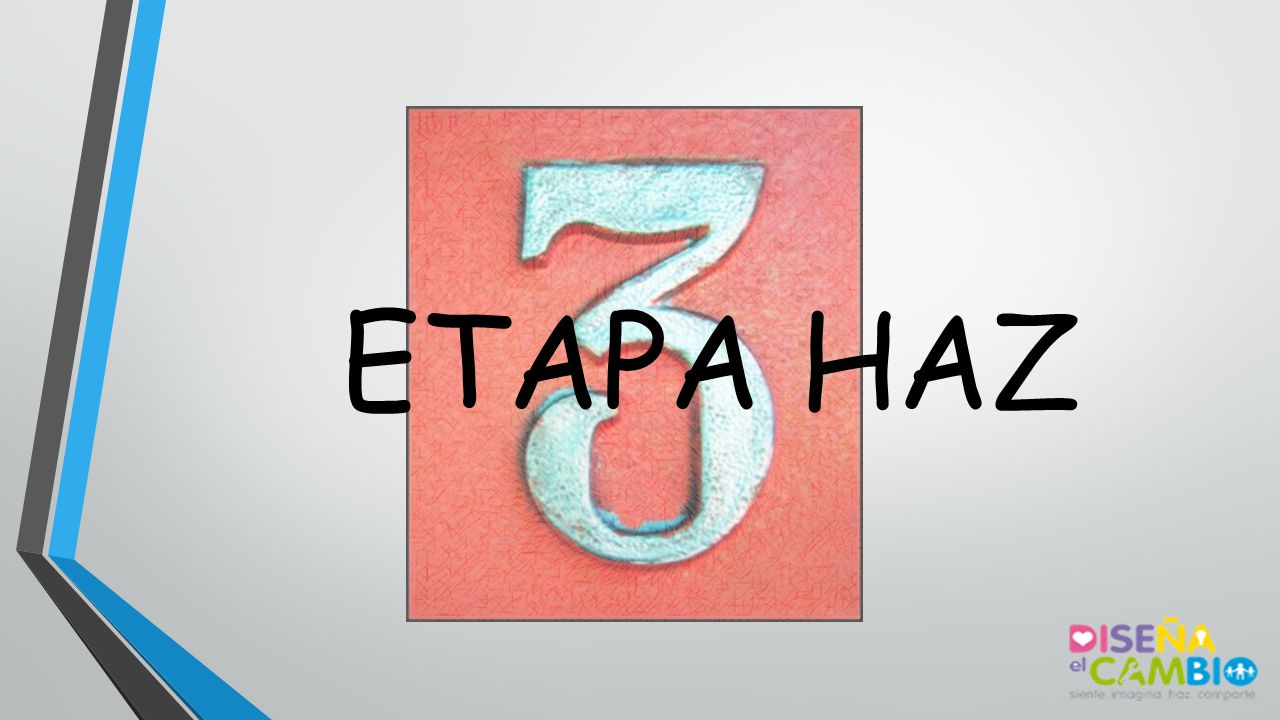In this image, the background is a light gray. Near the top left corner, two parallel lines—one black and one blue—descend at a slight angle, approximately 20 degrees, shifting slightly to the left. About 75% down the image, the lines change direction, angling to the right at around 30-45 degrees until they reach the bottom. Dominating the center of the image is an orange square with a subtle black outline. Inside this square is a white number 3 displayed in a medieval font. Above the number 3, the word "ETAPAZHAS" appears in a black, primitive-looking font. In the bottom right corner, there is additional text that reads "DISENIAL COMBIO," accompanied by a small blue circle logo depicting two parents holding children. This text is rendered in a very light brown-gray, making it barely visible.